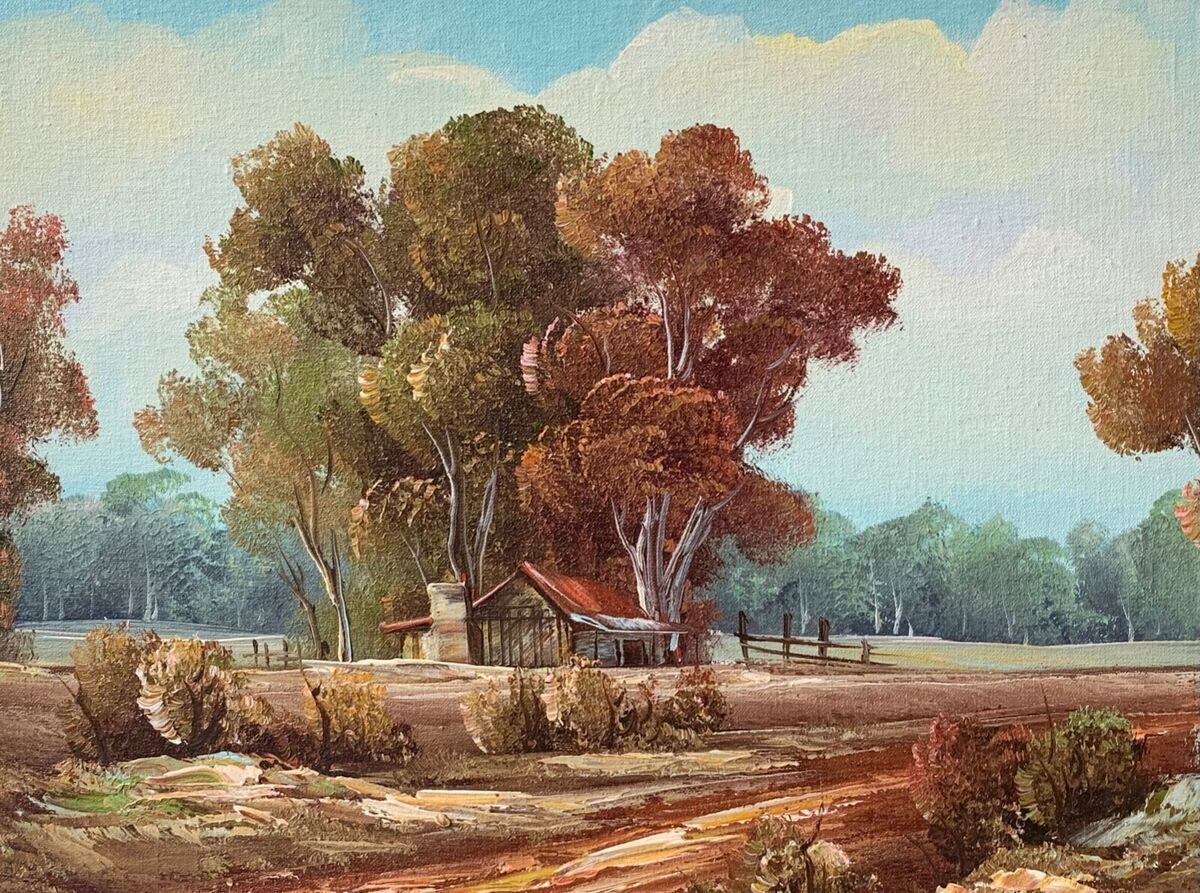This artwork depicts a charming, weathered house situated in a serene countryside setting. The house, with its distinctive red roof and side chimney, is framed by a lush backdrop of very tall trees, displaying a mix of red and green leaves, which accentuate the rural beauty. A large canopy adorns the front door, providing a welcoming entrance. Extending from both sides of the house are small wooden fences, adding to the rustic charm. In the foreground, numerous tan-colored bushes suggest the changing seasons. The scene is set under a blue sky with scattered clouds, amplifying the sense of tranquility. A vast forest stretches behind the house, enclosing it in nature's embrace. The overall palette of blues, greens, browns, and pastels enhances the painting's timeless and bucolic appeal.